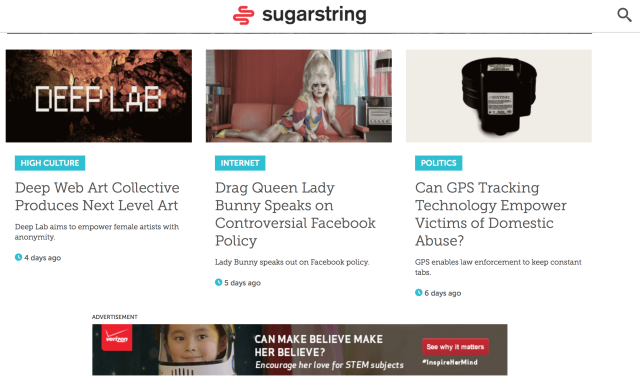**Image Description:**

The image features a white background with a red squiggly line prominently located in the center. Next to this line, black text reads "SugarString," written as one word. In the upper right-hand corner, there is an illustration of a magnifying glass. Below these elements, a black horizontal bar stretches across the image.

Underneath the bar, there is text surrounded by imagery resembling an underwater scene or cave with brown tones, contrasted by a predominantly black background. Superimposed in white text are the words "Deep Lab." Further below, in blue and white text, it reads "Deep Culture." Following this, black text states, "Deep Web Art Collection produces next-level art. Deep Lab aims to empower female artists with," and notes that this initiative began four days ago.

Adjacent to this, there is an image of a person with large blonde hair, identified as a drag queen named Lady Bunny, sitting on a white couch. In matching text style, it states, "Lady Bunny speaks out about Facebook policy" with an additional note that this occurred five days ago.

The image also presents a section with a grey background featuring a black device resembling a GPS tracking unit, typically used for individuals on parole. The accompanying text under the "Politics" section queries, "Can GPS tracking technology empower victims of domestic abuse?" followed by the statement, "GPS enables law enforcement to keep constant tabs," dated six days ago.

Additionally, there’s a screenshot of an Asian child wearing a space helmet. To the left of this image is the Verizon logo in white, and to the right, text reads, "Can make-believe make her believe?" with a mention of STEM projects.